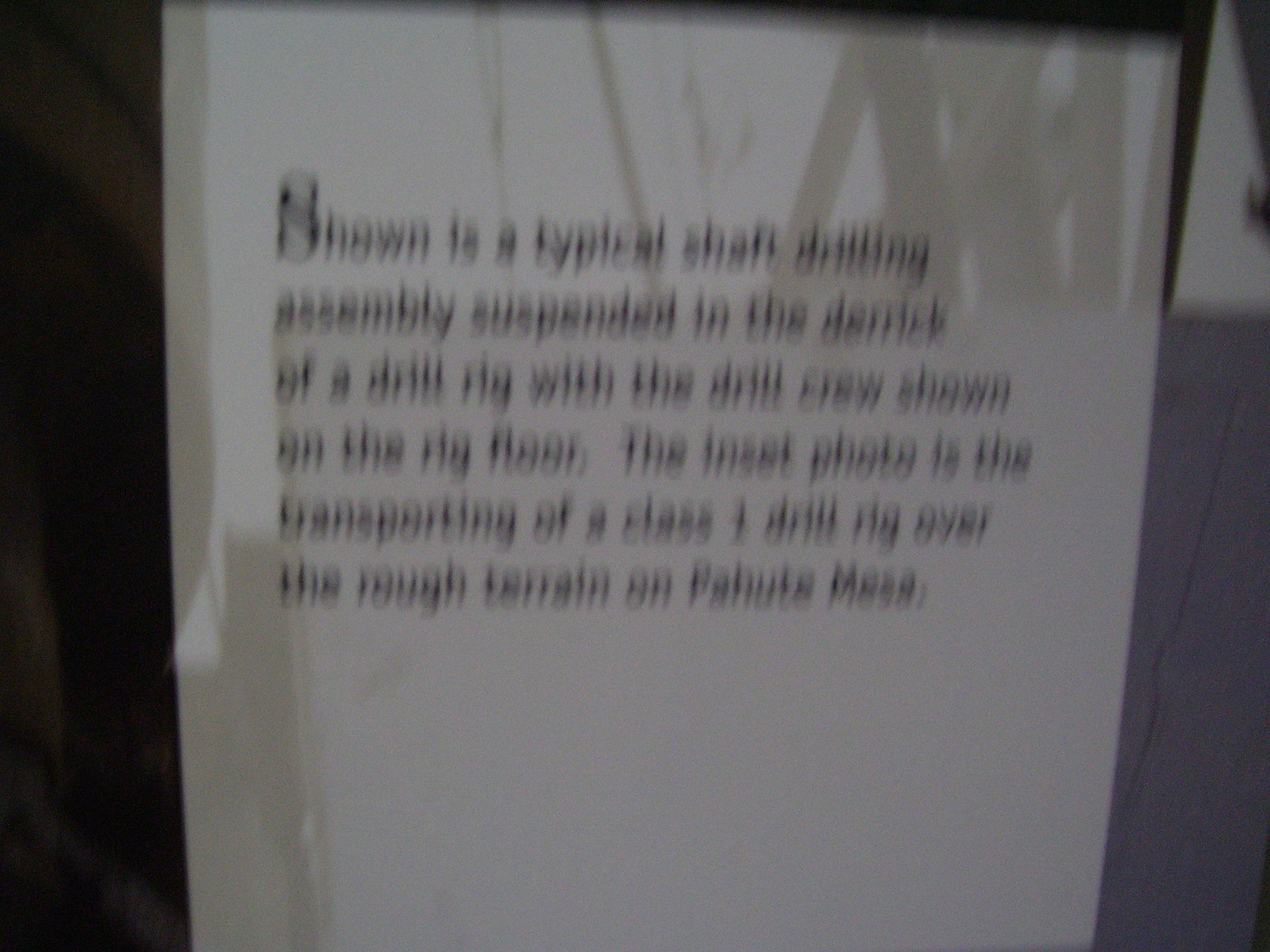A close-up photograph captures a piece of paper taped to the inside of a glass door. The paper contains a paragraph in black letters at the top, describing a typical shaft drilling assembly suspended in the derrick of a drill rig, with the drill crew visible on the rig floor. An inset image depicts a Class One drill rig being transported over rough terrain on Pahut Mesa. To the right of the paper, a gray wall or door is visible, and in the top right corner, the edge of another piece of paper can be seen. Reflected in the glass at the top of the image is the silhouette of a metallic structure in the background.